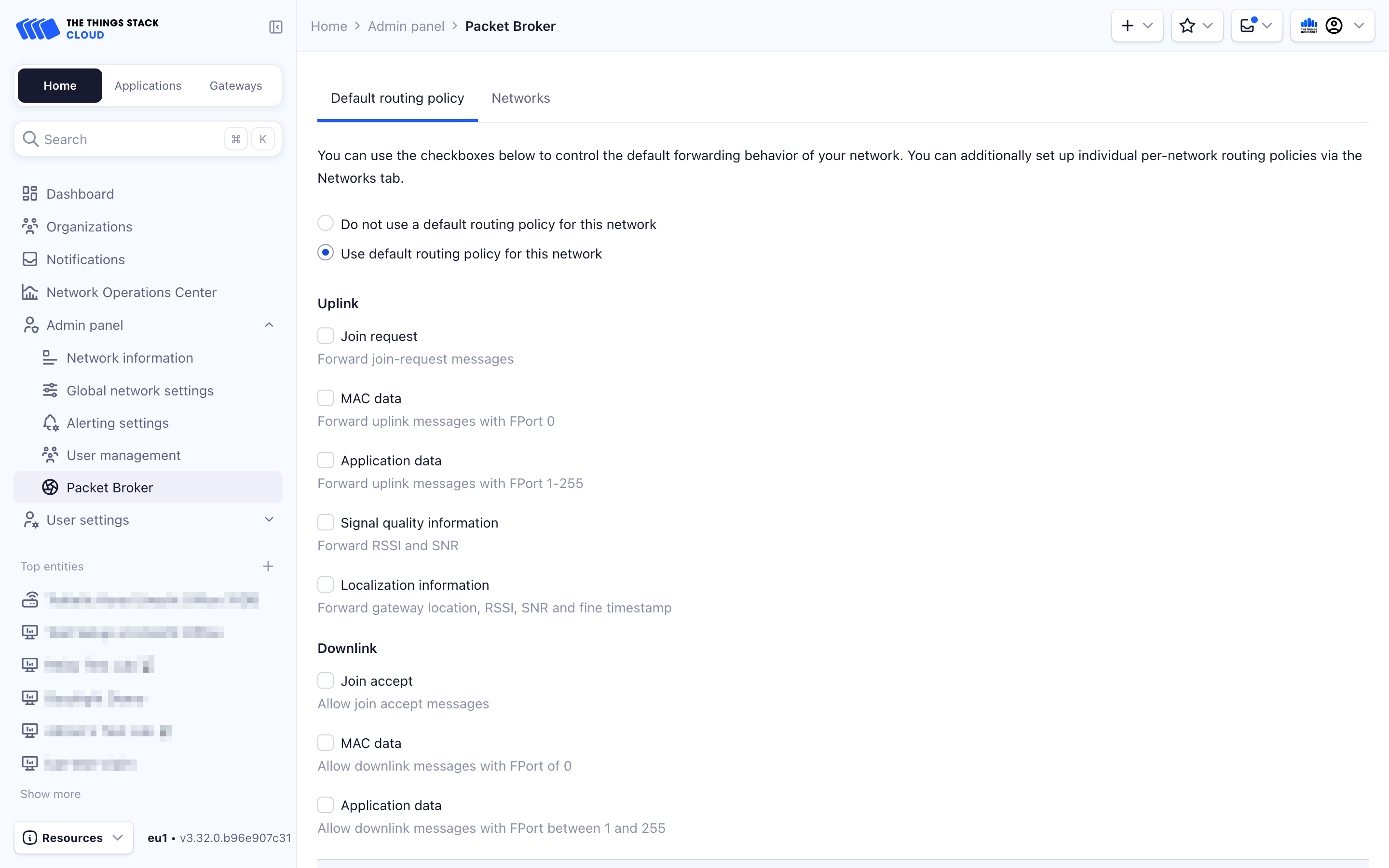**Caption:**

The image features a screen with an all-white background. In the upper-left corner, there are headers that read "General Information" and "Network Information." Below these headers, the screen appears to be displaying a network's routing policy settings. The specific details include:

- A gray-colored field labeled "ID" with the value "000013."
- Another labeled field for "Name," though the actual name is unspecified.
- Under "Network Contact Information," it records the "Last Policy Change" as January 7th, 2022 at 13:29.

The section for "Device Address Blocks" specifies a prefix of "2600::/7."

Routing policy settings include:
- "Set Routing Policy towards this network":
  - "Use default routing policy for this network"
  - "Use network-specific routing policy" (checked in blue).

Additional options for Uplink Join Request include:
- "Join before Join Request messages and MAC Data."
- Forwarding of uplink messages with "F port 0" is checked in blue.
- Forwarding of application data with "F port 1-255".

Furthermore, information regarding network metrics and localization features:
- Forward "RSSI" and "SNR" (checked in blue).
- Forward "Gateway Location," "RSSI," "SNR," and "Fine Timestamp" (checked in blue).